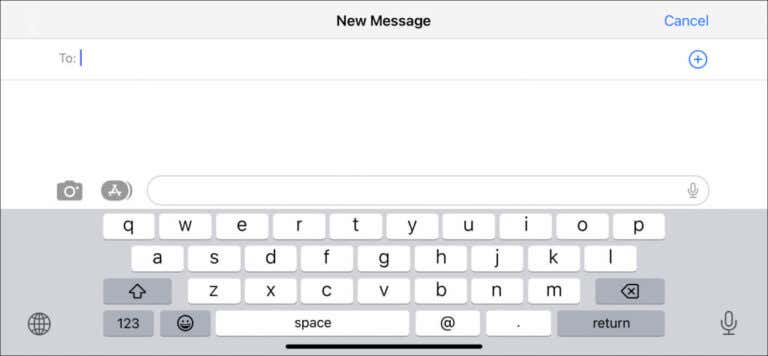The image displays a messaging interface. At the top, there is a header labeled "New Message" with a "Cancel" button situated to the right. Below the header, there is a "To:" field marked by the word "To" followed by a comma and a line where a recipient's name can be typed. To the left of this input field, there's a circular icon with a plus sign, indicating the option to add contacts to the message.

Under the "To:" field, there are several icons arranged horizontally. The first icon depicts a camera, followed by another icon which is not clearly described. Beneath these icons is a search bar equipped with a microphone icon on its right side, suggesting voice search capabilities.

The lower section of the image showcases a full QWERTY keyboard set against a gray background. At the very bottom left of the keyboard is a microphone icon, while the bottom right features a globe icon, typically used to change languages or input methods. Running nearly across the middle of the keyboard, a prominent black line is visible.

The interface is user-friendly and organized, indicating different functionalities available for composing a new message.